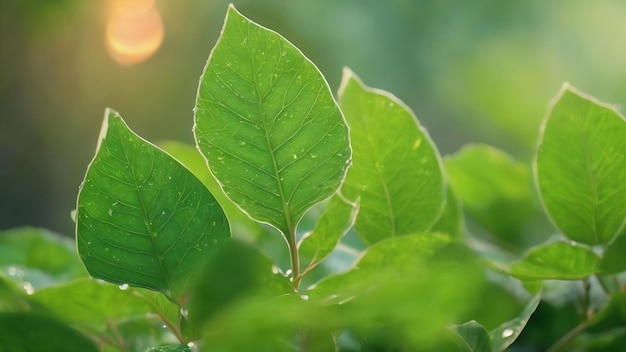This image is a close-up photograph of a vibrant green bush taken outside, likely just after a rain shower as evidenced by the droplets of water on the leaves. The leaves, which are oval or football-shaped with visible veins, dominate the central portion of the image, appearing slightly to the left and right towards the bottom middle. The entire photograph has a high-definition aspect ratio, making it wider than it is tall. A light source from the top left corner, casting an orangey hue, illuminates the scene, adding a slight warmth. The background is blurred, emphasizing the fresh and brilliant green leaves in the foreground. Additionally, there's a distinctive, small orange dot in the blurred upper left corner, contributing to the overall composition.